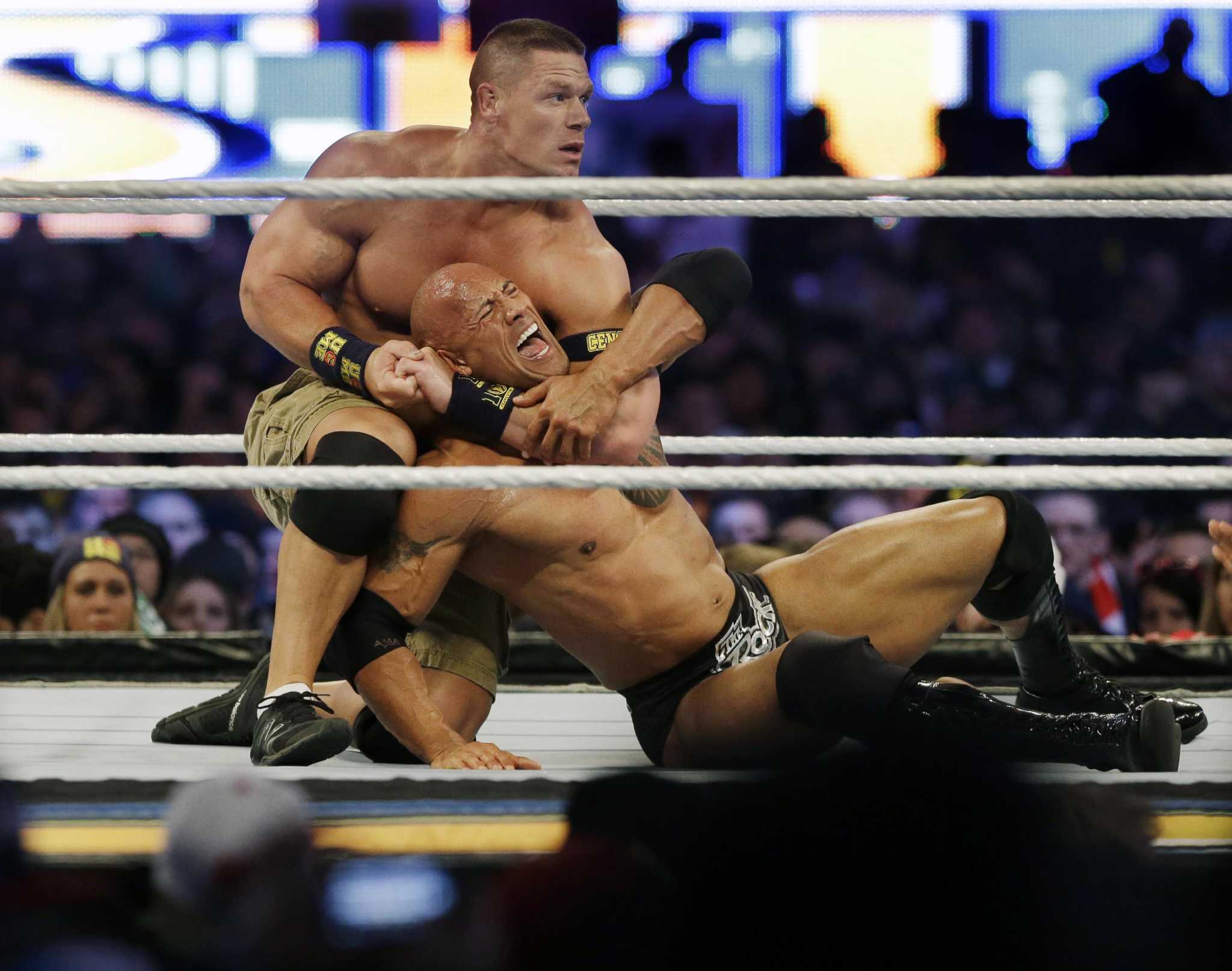This image is a detailed, colored still from a WWE wrestling match, capturing the intense moment between two iconic wrestlers, John Cena and The Rock. The shot is taken from a perspective just above ringside, providing a clear view of the white ropes enclosing the ring, which stretch horizontally across the image. The crowd forms a blurred backdrop at the top of the frame, with indistinct faces, colorful silhouettes, and various signs and lights.

Centered in the ring, John Cena, a light-complexioned, muscular wrestler with short brown hair, is on one knee, applying a firm headlock on The Rock. Cena is dressed in khaki shorts, black knee guards, short white socks, black sneakers, and wristbands with yellow accents. His clenched hands tightly grasp around The Rock’s neck, while he looks outward, seemingly at the referee.

The Rock, known for his dark complexion and bald head, appears to be in visible pain with his mouth open. He is seated on the ring floor, supporting himself with his right hand on the mat. His muscular build is showcased with black wristbands, black elbow bands, and a distinctive tattoo on his chest and arm. Dressed in minimal black wrestling shorts with white text near the crotch, black knee guards, and long black boots with black laces, The Rock’s left arm tries to counter the headlock around Cena’s left forearm. The ring floor beneath them is a light gray, contrasting the wrestlers' intense struggle in the spotlight.